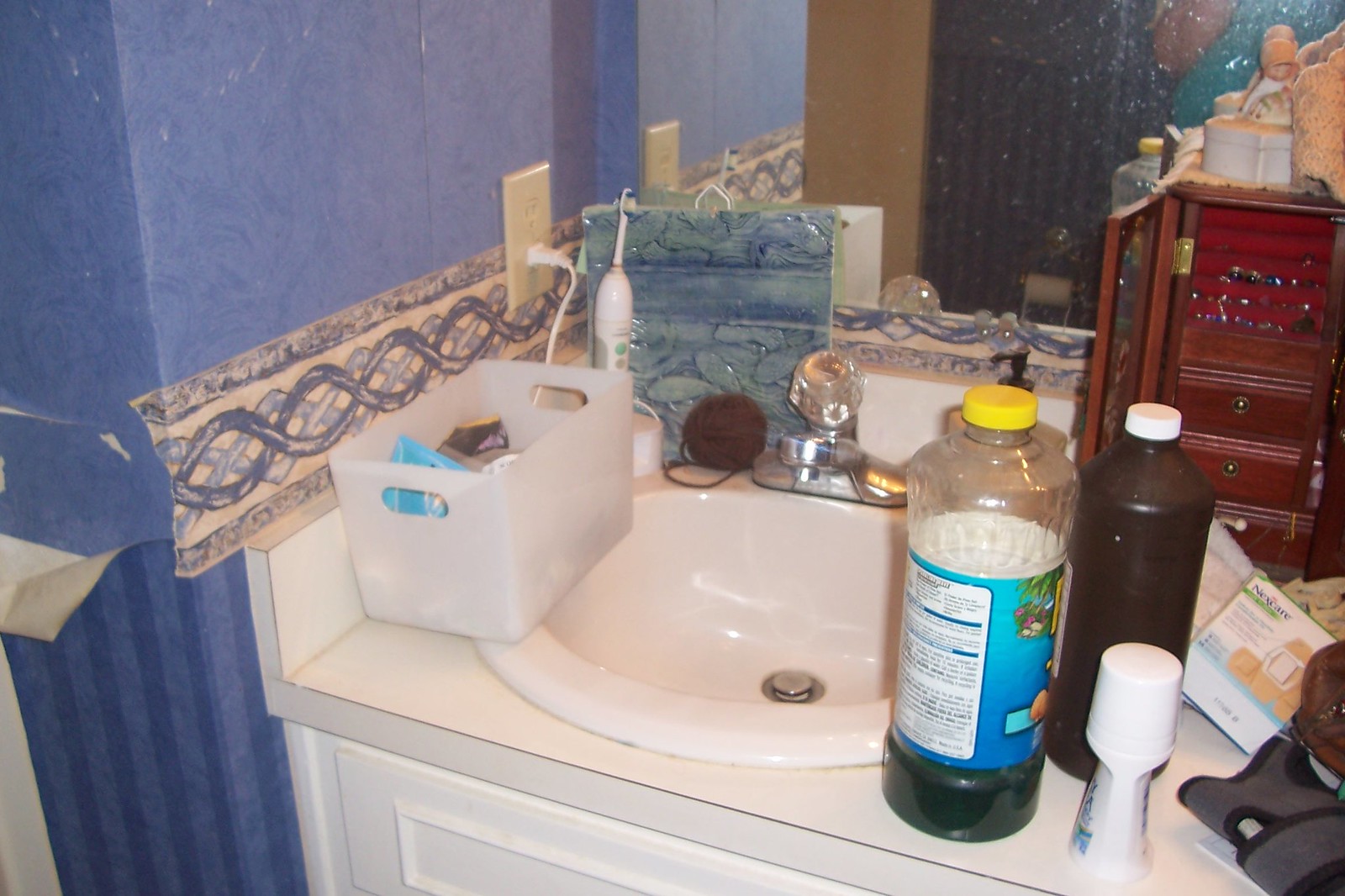The image depicts an extremely compact and cluttered vanity bathroom area. The sink counter is heavily crowded with various items. On the left-hand side, there's an electric toothbrush in front of a plastic basket filled with miscellaneous items. To the right of the sink are two containers: a clear one filled with blue liquid and a brown one, both accompanied by a deodorant holder. Against the wall, behind these items, stands a jewelry box that's piled with assorted clutter, including papers and a tape container. The left-hand wall is covered with poorly-torn, light blue wallpaper featuring a helix pattern trim. The overall scene exudes a sense of extreme disorganization and congestion.